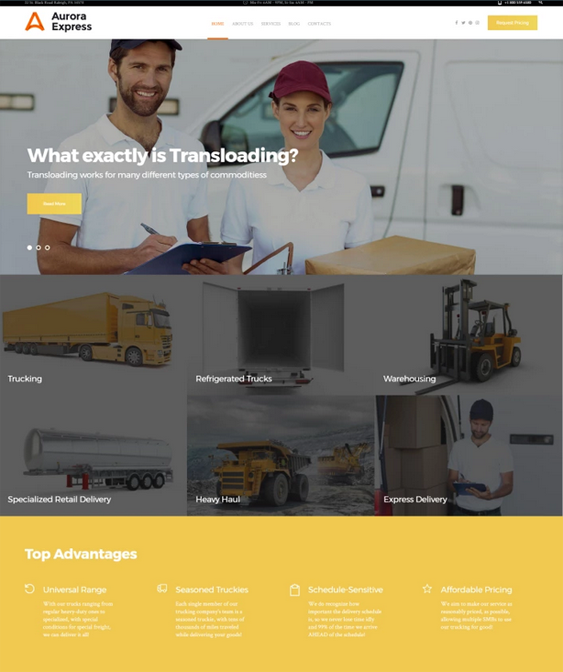The displayed image appears to be from a shipping website called Aura Express. At the top of the page, there is a distinctive dark yellow triangular logo pointing upwards with a curved base, accompanied by the text "Aura Express." In the top right corner, there's a rectangular button with a yellow background and white text.

Below the logo, a photograph showcases a man and woman standing in front of a white van. The man, who has a dark tan and a beard, is dressed in a short-sleeve blue polo shirt and a matching blue hat. He holds a pen and a blue clipboard. Standing to his right, the woman is smiling at the camera. She wears a maroon hat and a white short-sleeve polo shirt and holds both a clipboard and a brown package.

Further down the page, a grid of images is displayed, organized into two rows and three columns. In the first row, the image on the left is labeled "Trucking" and depicts a yellow tractor-trailer. The middle image is captioned "Refrigerated Trucks" and shows an open white trailer. The right image, labeled "Warehousing," features a yellow and black forklift.

In the second row, the left image is labeled "Specialized Retail Delivery" and portrays a silver cylindrical trailer. The middle image, titled "Heavy Haul," shows a dump truck operating in a mine. The right image, labeled "Express Delivery," features a man in a blue cap and white polo shirt holding a clipboard next to a van loaded with boxes.

Additionally, there is a section with a yellow background and white text labeled "Top Advantages." This section lists four columns with the following headers: "Universal Range," "Season Truckees," "Scheduled Sensitive," and "Affordable Prices."